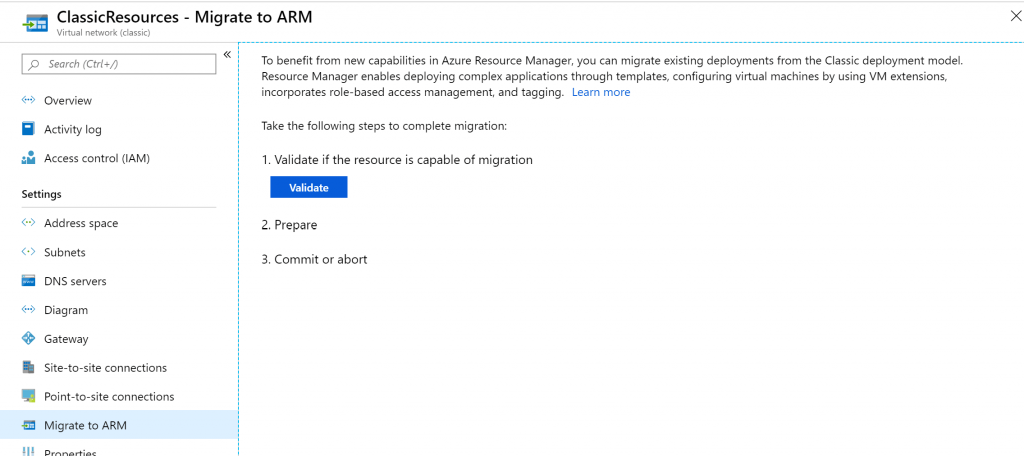Screenshot of the "Migrate to ARM" Section in Azure Portal

The screenshot displays the "Classic Resources, Migrate to ARM, Virtual Network Classic" section at the top left of an Azure portal interface. Below this, a vertical menu lists multiple navigation options: Search, Control Plus Slash, Overview, Activity Log, Access Control (IAM), Settings, Service Space, Subnets, DNS Servers, Diagram, Gateway, Site-to-Site Connections, Point-to-Site Connections, Migrate to ARM, and Properties.

To the right, detailed instructions on migrating from the Classic Deployment Model to Azure Resource Manager (ARM) model are provided. The text emphasizes the benefits of the ARM model, such as deploying complex applications through templates, configuring virtual machines using VM extensions, and incorporating role-based access management and tagging. Additionally, there is a call to action to learn more about these capabilities.

The migration steps are outlined as follows:
1. Validate if the resource is capable of migration. (This step is accompanied by a blue rectangular button labeled "Validate.")
2. Prepare.
3. [Step 3 is missing in the description].
4. Commit or Abort.

Note: The image is purely textual with no photographic elements or images of people included.